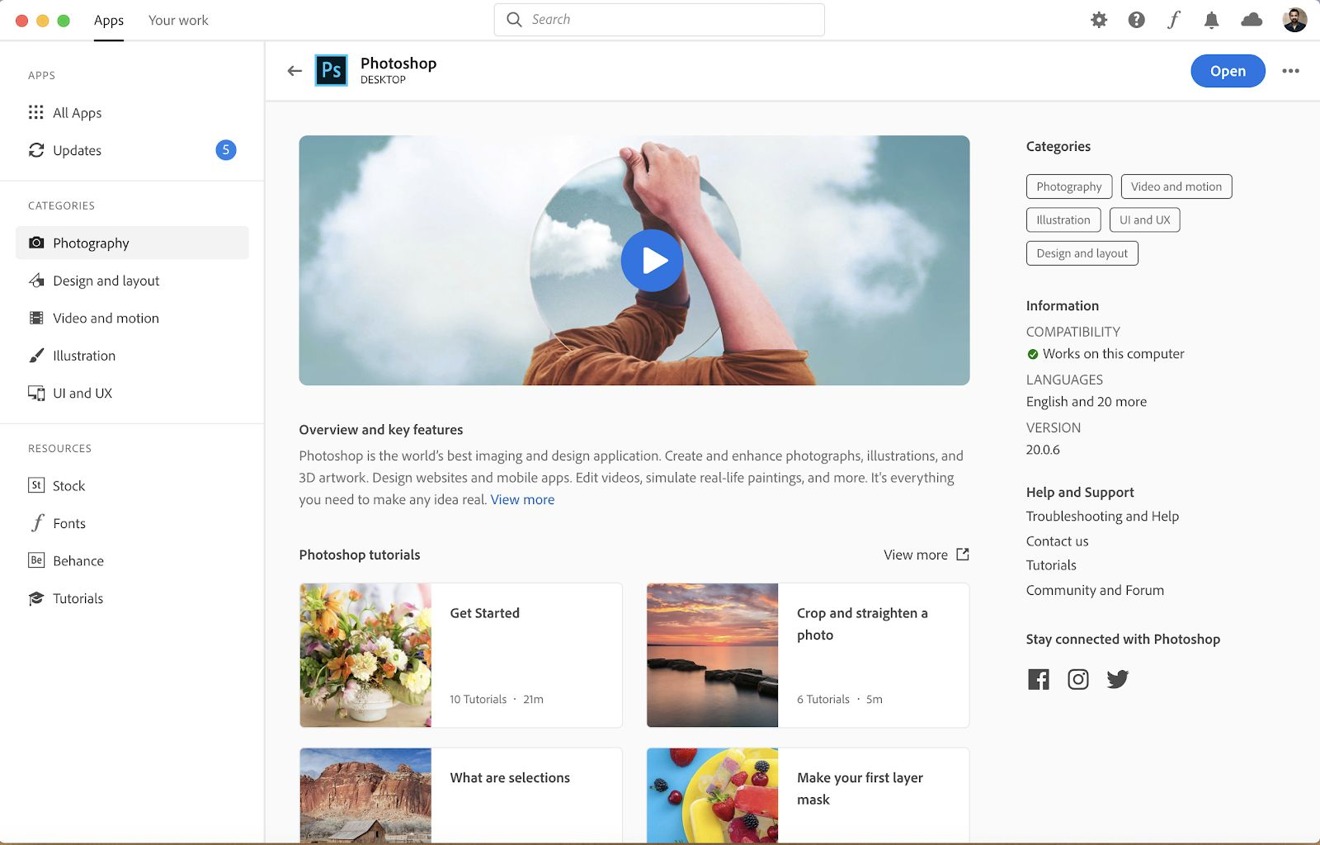This image is a screenshot from a computer screen displaying the Photoshop interface. At the top, it clearly shows the title "Adobe Photoshop" alongside an icon featuring a "P" in a box next to an "S" and an arrow pointing to the left, indicating navigation options. In the upper right corner, there is a prominent blue button labeled "Open" in white text.

Below this header section, the main content area features a partially visible photograph of a person. The person appears to be raising their arms over a spherical object, likely a globe, while wearing a beige sweater. The background depicts a blue sky with scattered white clouds, creating a serene and uplifting atmosphere. 

Accompanying the image is an informational text block titled "Overview Key Features." The text describes that "Photoshop is the world's best imaging and design application." It continues to explain that users can "create and enhance photographs, illustrations, and 3D artwork," as well as "design websites and mobile apps." 

Towards the bottom of the screen, there are additional resources, including Photoshop tutorials designed to help users learn and navigate the software effectively.